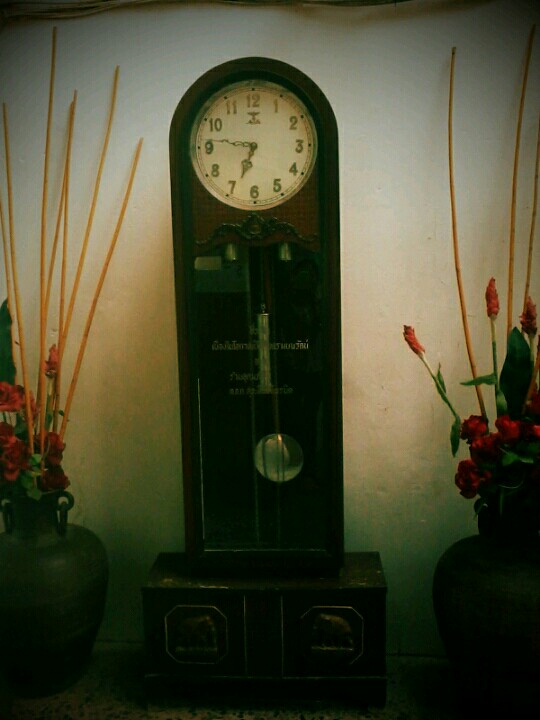In a dimly lit room with a backdrop that appears grayish due to the shadows, the main focus is a stately grandfather clock. The clock stands on a black or dark-colored pedestal, embellished with intricate elephant engravings. A golden pendulum swings within the glass-case center, while the top showcases a white clock face adorned with ornate hour and minute hands, and dark-colored metal numerals. Flanking the clock are two large vases or pots, possibly black or dark green in color, each containing an arrangement of roses and other flowers. The mix includes vibrant red blooms, green stems, and notable yellow sticks, adding a touch of color against the muted background.